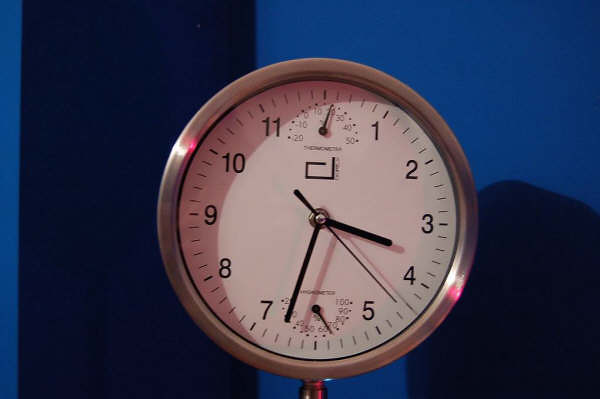A close-up photo showcases a round clock encased in stainless steel, seemingly resting on its winding button or a stand. The clock face is white, featuring black numerals and minute markers. The hour and minute hands are straight, black lines, while a thin black needle serves as the second hand. An additional circle at the bottom of the clock face contains a smaller black needle, labeled "hygrometer" across the top. The background transitions from royal blue on the left to a darker navy blue on the right, likely due to the clock's shadow. A bright light highlights the clock, casting a crescent-shaped shadow on its face.